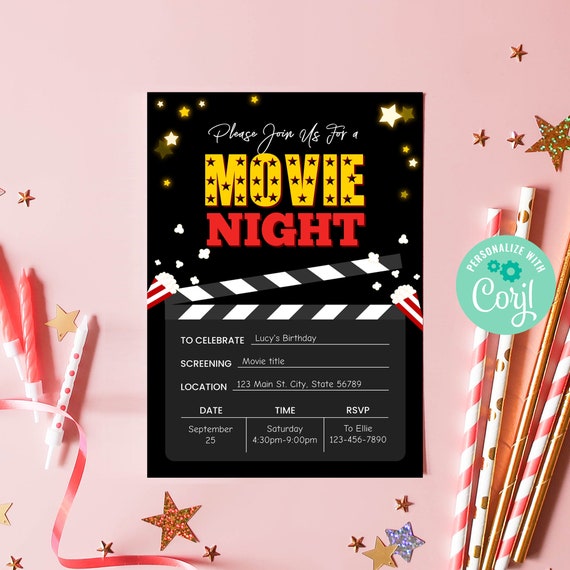The image showcases a stylishly arranged product photo, set against a pink background. At the center is a black invitation poster for a movie night to celebrate Lucy's birthday, featuring placeholder text: "Please join us for a movie night to celebrate Lucy's birthday. Screening [Movie Title]. Location: 123 Main Street, City, State, 56789. Date: September 25th. Time: 4:30 p.m. to 9:00 p.m. RSVP to [123-456-7890]." The poster is surrounded by decorative elements including white birthday cake candles with pink dots on the left, glittery stars in gold and purple, and pink and gold straws on the right. A teal circle at the top right is superimposed with the word "personalized," although the exact text after "Coral" is partly obscured, resembling "CORYIL." The aesthetic suggests a digitally enhanced presentation, capturing a blend of elegance and festive charm with colors like pink, black, gold, and silver.